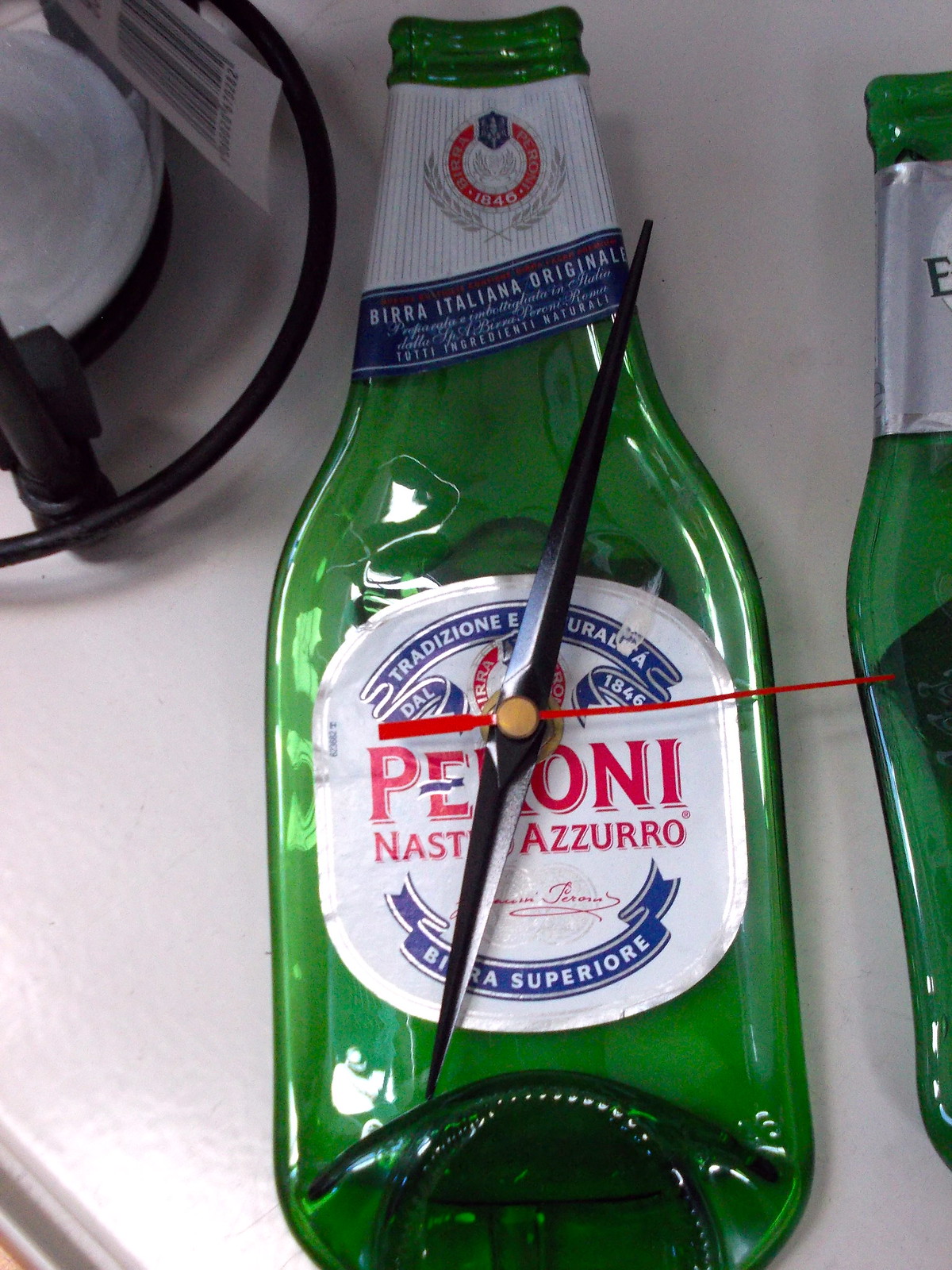This captivating image showcases a flat, green glass bottle, seemingly repurposed into a clock. The base of the bottle appears deliberately crushed, adding character to its unique form. At the top of the bottle, a white label prominently displays "Peroni" in bold red letters, enclosed by a red circle. Surrounding this is a blue label bearing the inscription, "Birra Italiana Originale," indicating its Italian origins. The clock mechanism is integrated seamlessly, with black hour and minute hands, and a red second hand. Notably, there are no digits on the bottle clock, lending it a minimalist yet intriguing aesthetic. The bottle's surface features text in another language, enhancing its exotic and vintage appeal.